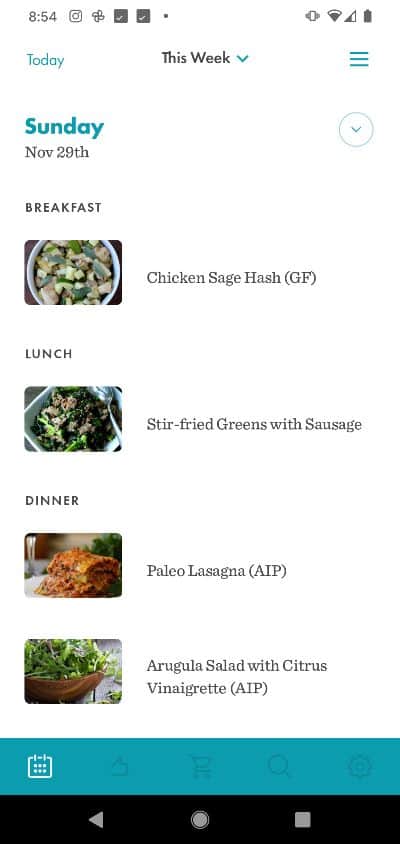This is a detailed screenshot of a cell phone interface displaying a meal planning app against a white background. 

**Top Status Bar:** 
- The time is shown as "8:54" in black text.
- Icons displayed from left to right include a camera icon, a Google Photos icon, two black checkboxes with white check marks, and a large black dot.
- On the right side, there are icons for a phone signal, a Wi-Fi signal (showing 2 out of 4 bars), and a fully charged black battery icon. Below the battery icon are three horizontal turquoise blue lines stacked atop one another.

**Calendar Section:**
- In the center, the date section highlights "This Week" in bold black text with a blue down arrow to its right.
- To the left, it says "Today" in blue text.
- Beneath, it specifies "Sunday, November 29th" in bold blue text, paired with a blue circle and blue down arrow on the right.

**Meal Plan:**
- Under the date, there is a label for "Breakfast" in black text with a thumbnail image of a bowl containing food. To the right, it specifies "Chicken Sage Hash."
- The next label, "Lunch," features a thumbnail image of greens in a square white bowl. On the right, it indicates "Stir-Fried Greens with Sausage" in gray text.
- Following that, "Dinner" is labeled with an image of a piece of lasagna. To the right, it reads "Paleo Lasagna."
- The final item at the bottom is labeled "Arugula Salad with Citrus Vinaigrette." The left thumbnail shows a wooden bowl filled with greens.

**Bottom Menu and Navigation:**
- At the very bottom of the image, there is a horizontal turquoise bar. On the left-most end is a white calendar icon, followed by very faded light gray icons, possibly including a reload button, a square icon, a magnifying glass, and a round circle icon towards the right.
- Below this bar, on a black background, are navigation icons: a gray back arrow, a gray circle (likely the home button), and a gray square on the right.

This detailed description captures all elements present in the screenshot, including crucial visual details and textual information.